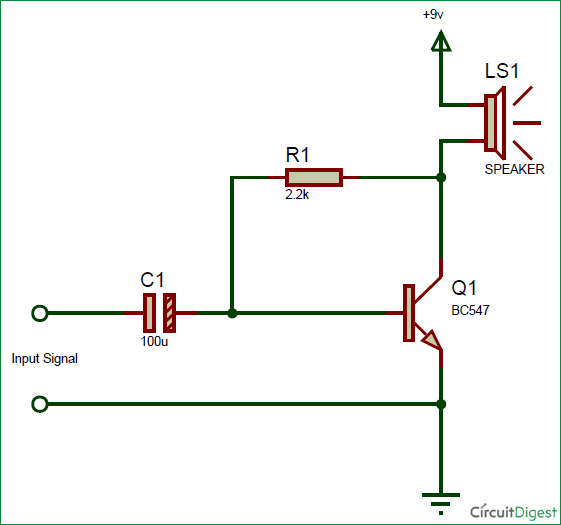The image is a detailed circuit diagram enclosed within a square green border. In the lower right corner, the label "Circuit Digest" appears, with "Circuit" in grey and "Digest" in green text. The diagram itself features green lines representing wires and various red and grey rectangular components within the circuit. The input signal is depicted on the left side as two green lines, branching out and connecting to several circuit elements labeled with specific functions and values, such as "R1 2.2K." On the upper right, there is a labeled speaker icon "LS1" with red lines indicating signal paths, suggesting the circuit’s output. Above the initial point of the circuit is a symbol with "plus NV," adding further complexity to the design. The overall layout maps out the electrical connections and components in a clear and structured manner, illustrating the flow and function of the circuit from input to output.